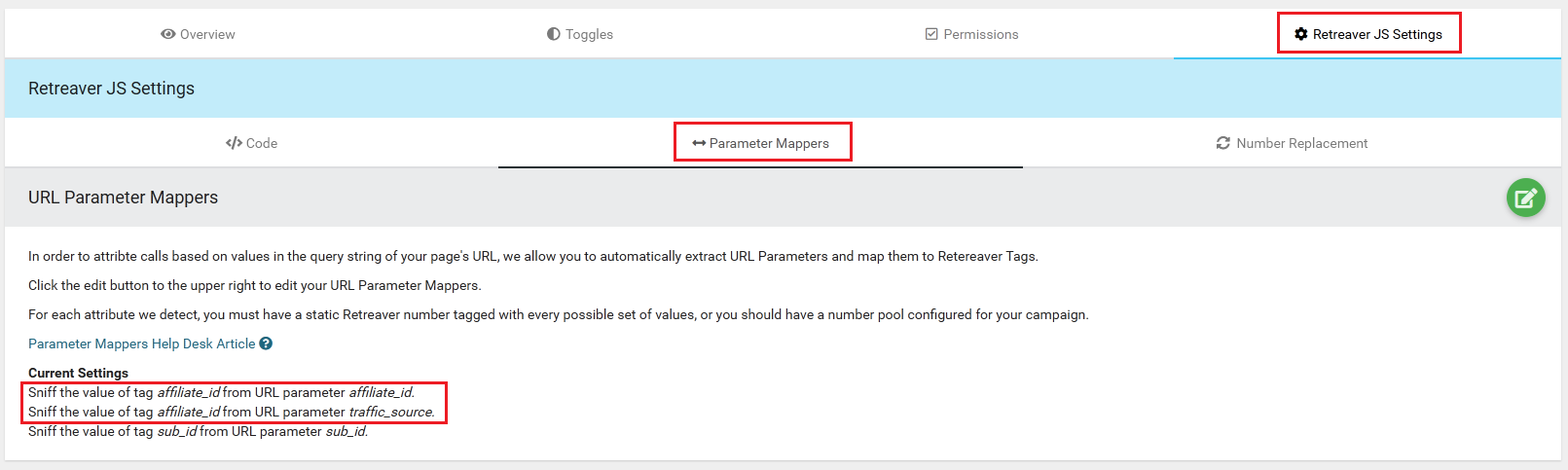Screenshot of a computer screen showcasing a web interface. At the top left, there is a label reading "Overview" next to another label "Toggles." Below them in the middle, it reads "Permission" alongside "Retriever JS Settings," both situated within a white rectangle with a red border, making it stand out prominently. Beneath this, there's a narrow blue rectangular box labeled "Retriever J Settings." Moving further down, there is a section titled "Code," followed by "Parameter Mappers," and "Number Replacement," with "Parameter Mappers" also enclosed in a red-bordered rectangle. Directly below that, "URL Parameter Mappers" is noted, ending with a green circle. The last segment contains detailed text explaining the procedure for attributing cause based on query string values in the page's URL. It mentions an automatic method for extracting URL parameters and mapping them to retriever tags, with additional information available via a help desk article. A particular instruction is highlighted within a rectangle, directing users to "sniff the value of tag affiliate ID from URL parameter affiliate ID."